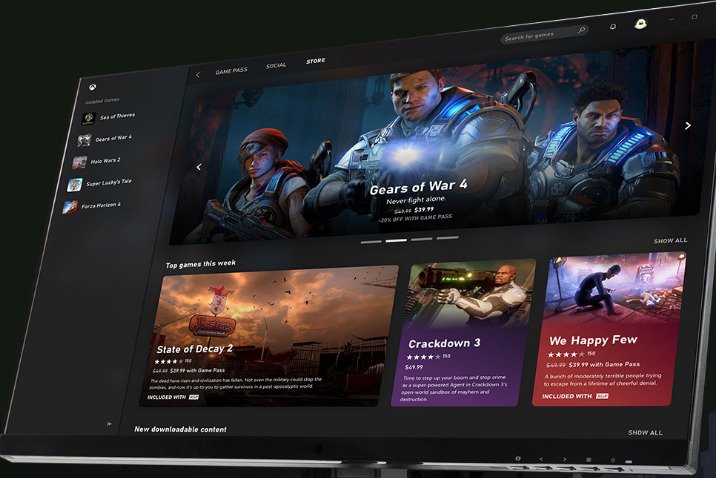In this image, the screen displays key visuals from four different video games against a predominantly black background. 

On the top left, "Years of War 4" features three armored characters – two men and one woman – equipped with flashlights. 

Next to it, "State of Decay 2" showcases an ominous sky filled with menacing clouds. 

"We Happy Few," positioned beside that, highlights a character clad in armor wielding a rocket launcher. 

Lastly, "Crackdown 3" depicts a dynamic scene where a character stands atop a brightly illuminated building, casting light into the night.

Along the left side, a white section displays additional text and icons relevant to the context. At the bottom of the screen, a silver line contains various buttons on the left side. The top right corner shows a settings wheel and a search bar, with the word "Store" prominently displayed in the center. 

The entire scene is set against a black background, creating a stark contrast that emphasizes the colorful and detailed game visuals.